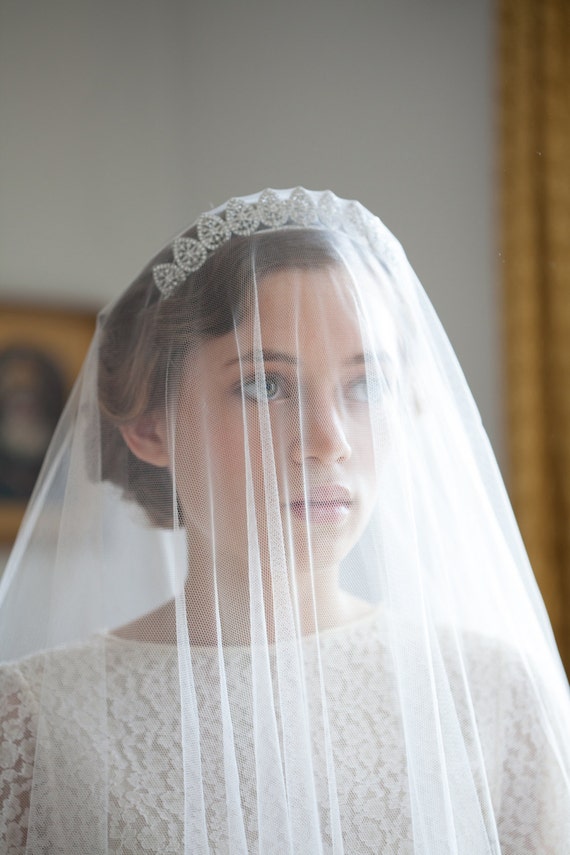This photograph features a bride adorned in a white lace dress with intricate floral detailing. She is wearing a white veil that partially conceals her face, complementing her elegant, wavy updo hairstyle. Her brown hair is elegantly styled to highlight a tiara with a teardrop design embellished with sparkling elements at its center. The bride's facial features are delicate, characterized by brown eyebrows, a well-defined nose, and soft, delicate lips. In the background, there's a white wall which is partially adorned with a piece of artwork that incorporates shades of brown, black, gold, and off-white. Additionally, a gold object is visible on the other side of the image, adding a touch of warmth to the scene.